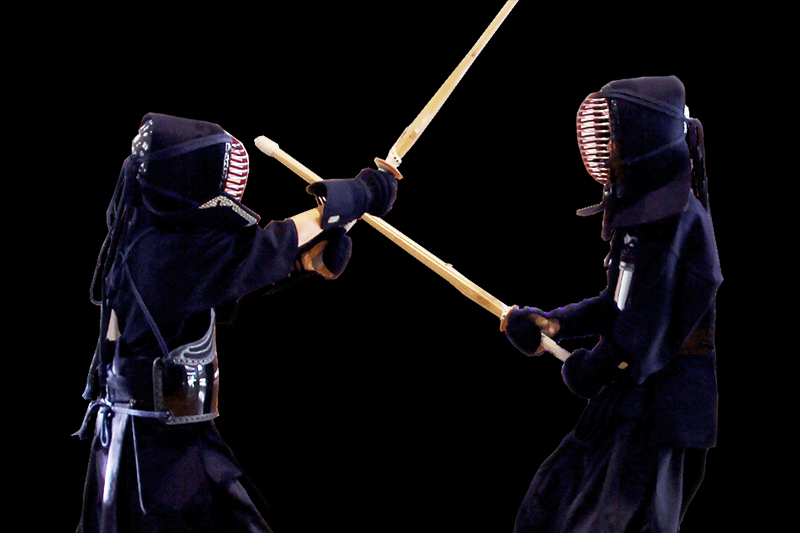This photograph captures two individuals engaged in the martial art of Kendo, facing each other in a poised duel amidst a stark black backdrop. Both practitioners are clad in traditional blue Kendo uniforms, complete with padded hand protection and protective guards around their torsos. Each wears a distinctive metal mask with horizontal bars, secured with blue strings tied at the back, to shield their faces. They hold large wooden swords aloft, with the figure on the left raising their sword high while the figure on the right extends theirs forward from the chest. The light brown shawls they've draped around their shoulders interact dynamically, adding fluid motion to the scene. The intensity of their stances, coupled with the solid black background, accentuates their focused confrontation.